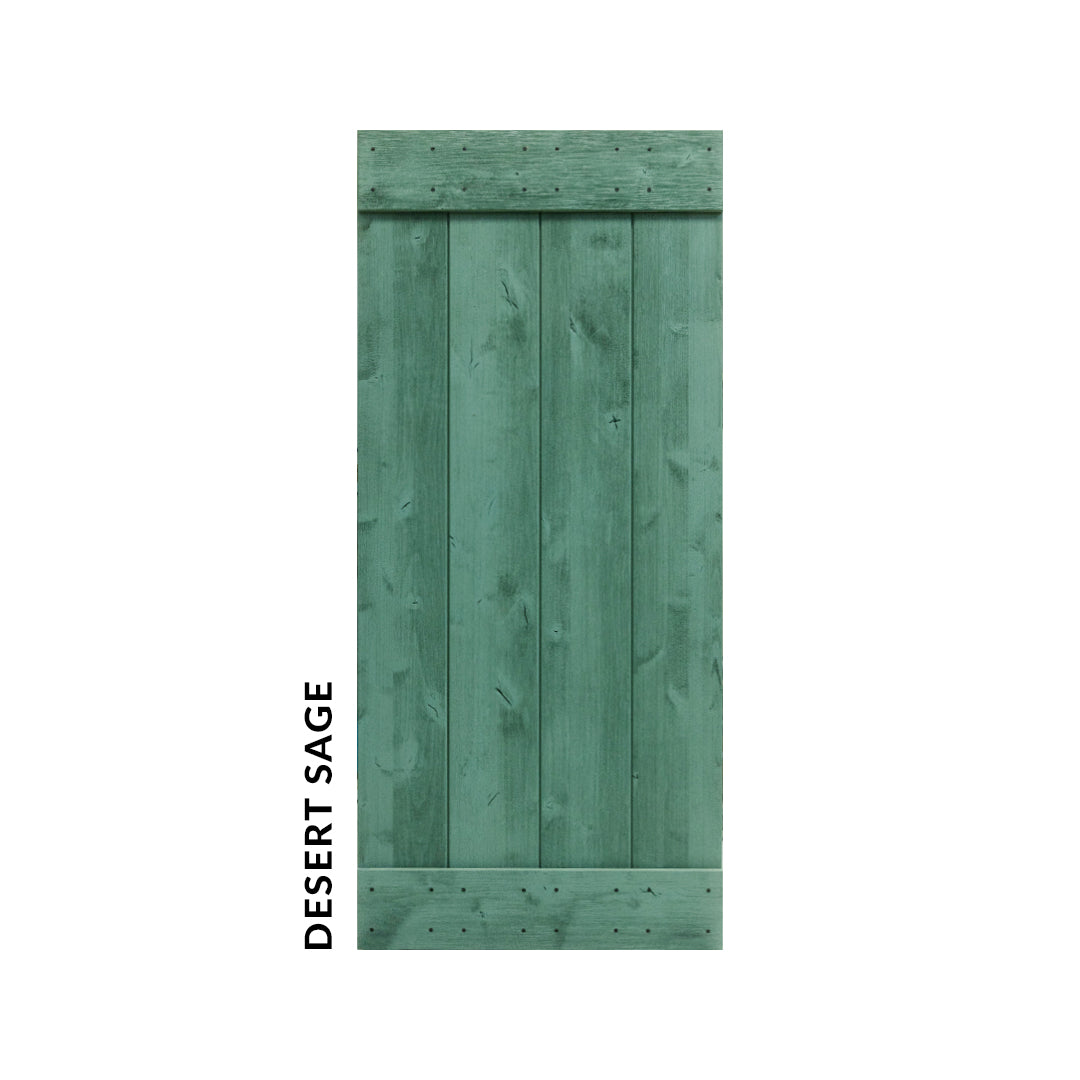The image is a photograph likely sourced online from a site dealing with paints or wood stains. It features a rustic wooden panel with a white background. The vertical paneled wood, which has a distinctive weathered texture, shows four vertical strips, each showcasing a light sage green tint with darker green grains and scratches. The horizontal top and bottom strips of the panel have visible nails and dots, adding to the rustic appearance. Along the left side of the image, the text "DESERT SAGE" is displayed in uppercase black letters positioned vertically. The interplay of the faded green hues and the distressed wood grain lends the panel an antique, earthy charm.